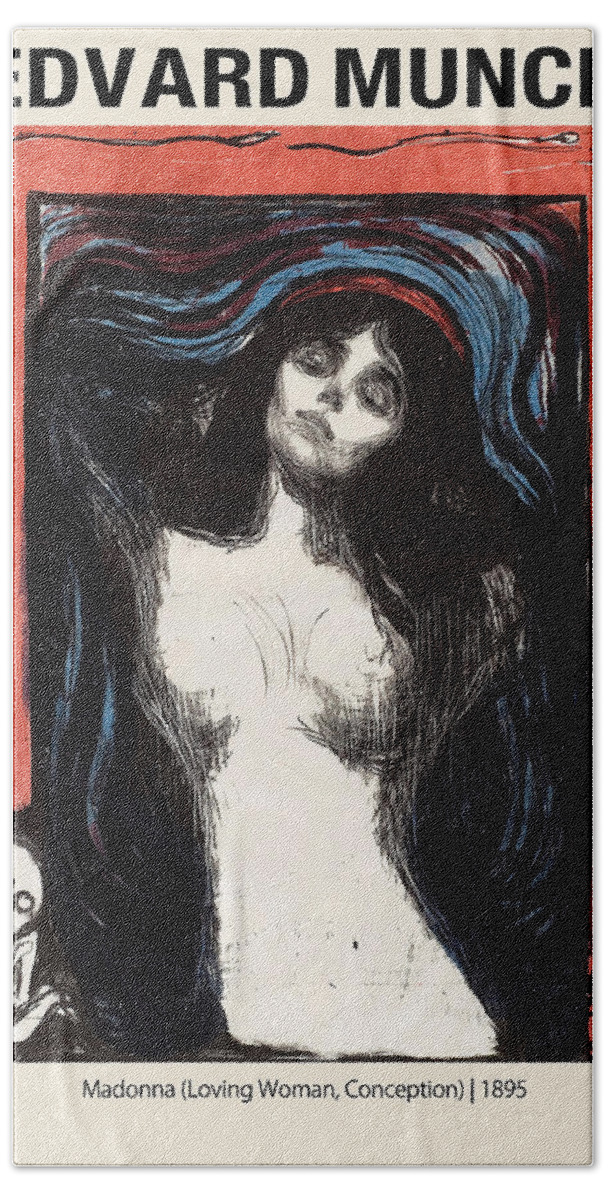This image is a vertically-oriented reproduction or print of a painting by Edvard Munch, titled "Madonna (Loving Woman, Conception)" and dated 1895. The top section of the image features the partially obscured name of the artist, Edvard Munch, against a gray bar background. The lower portion features the title and date in small, dark text. The artwork itself depicts a young, nude woman, viewed from the torso up, with a face rendered in a realistic style. Her dark, flowing hair melds into abstract swirls of black, blue, and red hues, which dominate the background, creating a dreamy and almost wave-like effect around her, evoking a sense of ethereal beauty.